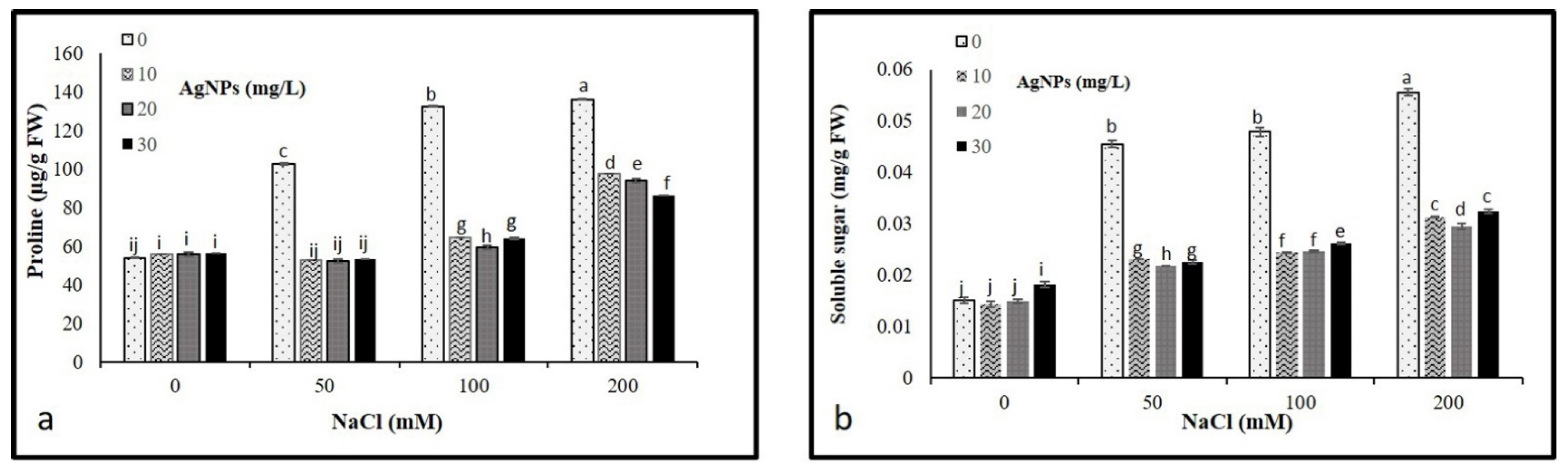The image consists of two side-by-side bar graphs labeled A and B. Each graph features four bars representing different concentrations of NaCl: 0, 50, 100, and 200 mM. The bars are differentiated by various patterns—speckled, lined, gray, and solid black. 

In graph A, the x-axis is labeled "Proline (mg/g FW)," while graph B has "Soluble Sugar (mg/g FW)" as its x-axis label. Both graphs share a y-axis scale, although the values differ slightly: graph A ranges from 0 to 160, and graph B scales from 0 to .6. The bars display varying heights indicating different data points, with some subtle differences in height between the corresponding sets of bars in the two graphs.